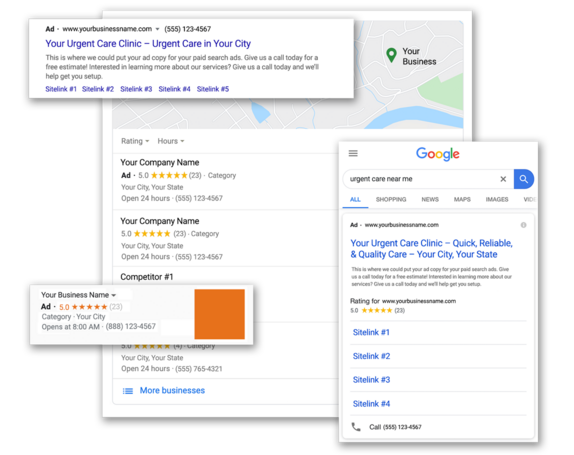**Detailed Caption:**

This image is a detailed montage of various screenshots from Google, prominently showcasing a Google business page template. The largest screenshot highlights this template, designed to provide prospective customers with an overview of how a business page could visually appear. It can be inferred that the company responsible for the montage specializes in offering services to businesses to enhance their online marketing strategies.

In the showcased template, instead of actual business details, placeholders such as "Your Business" are used. The template emulates the layout of authentic Google business pages, complete with features like a mock map in the upper right corner, which also says "Your Business". Beneath this, placeholders replicate the typical format seen in search engine results, listing "Your Company Name" with five gold stars, a category, city, state, a notice that the business is "Open 24 hours", and a dummy phone number.

Overlaying the top of the template is a banner illustrating an ad format on a Google search page. This section includes text akin to what a paid search ad might display: "Your Urgent Care Center - Urgent Care in Your City." Following this, it features a placeholder for ad copy, encouraging users to "Give us a call today for a free estimate. Interested in learning more about our services? Give us a call today, and we'll help you set up."

In the lower right corner of the montage, there's an additional mock-up presenting what a Google search results page would look like on a mobile phone. The search term entered is "Urgent care near me," showcasing how an ad might appear at the top of mobile search results, further emphasizing the practical application of these marketing tools.